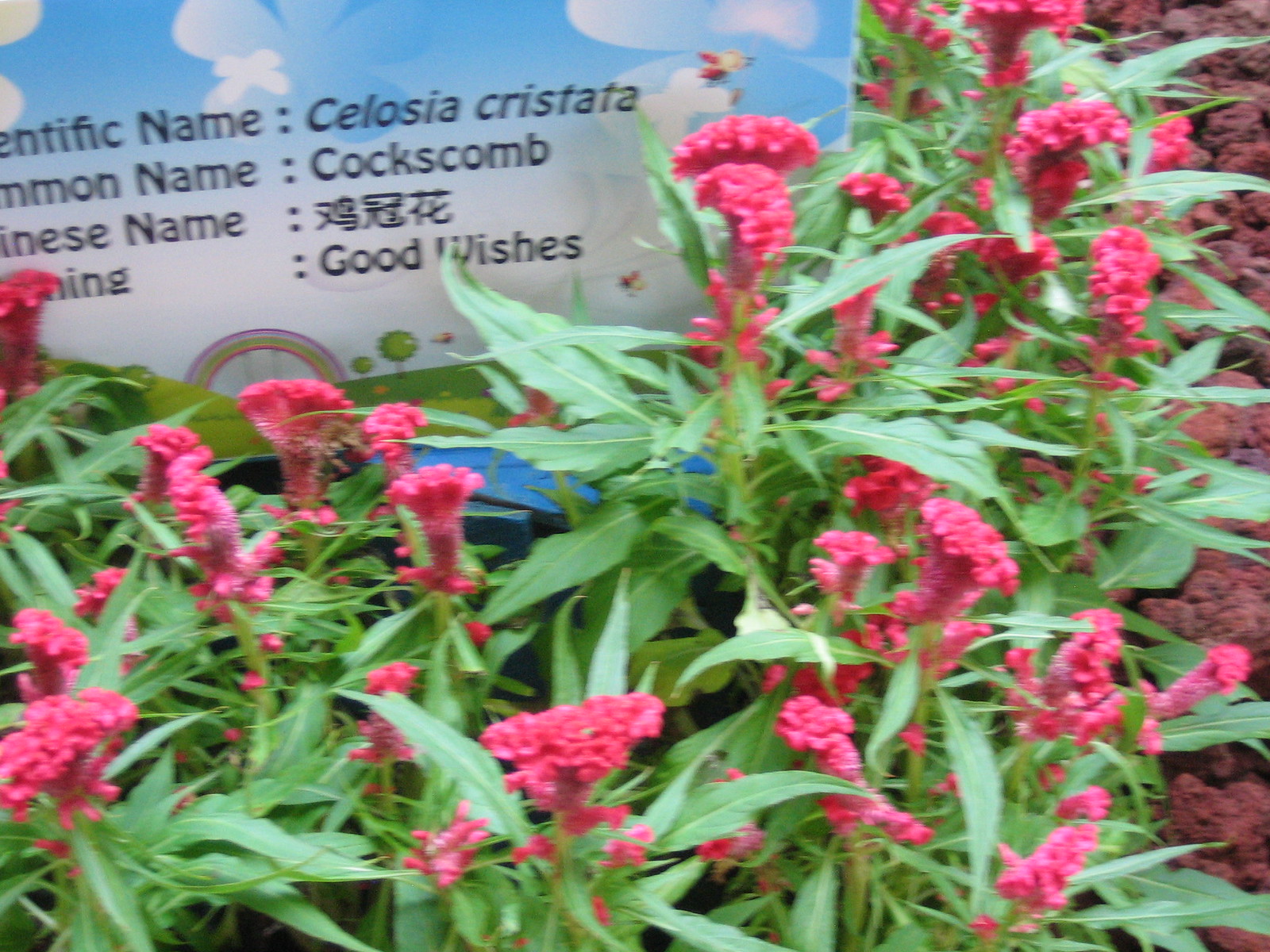This photograph, taken in a garden during the day, captures a patch of vividly colored flowers amidst a slightly blurred background. The primary focus is on the spear-shaped green foliage, similar in hue to typical lawn grass, with striking, clumped, and fuzzy flowers that range in color from pinkish to magenta to hot pink and red. Positioned prominently within this floral bed is a blue sign adorned with white cloud-like designs and black text. Although partially obscured, the sign clearly states the scientific name "Celosia cristata," the common name "coxcomb," the Chinese name written in characters, and the phrase "good wishes." To the right of the flowers, there is a reddish-brown ground covering, perhaps mulch or lava stones, further accentuating the captivating scene.